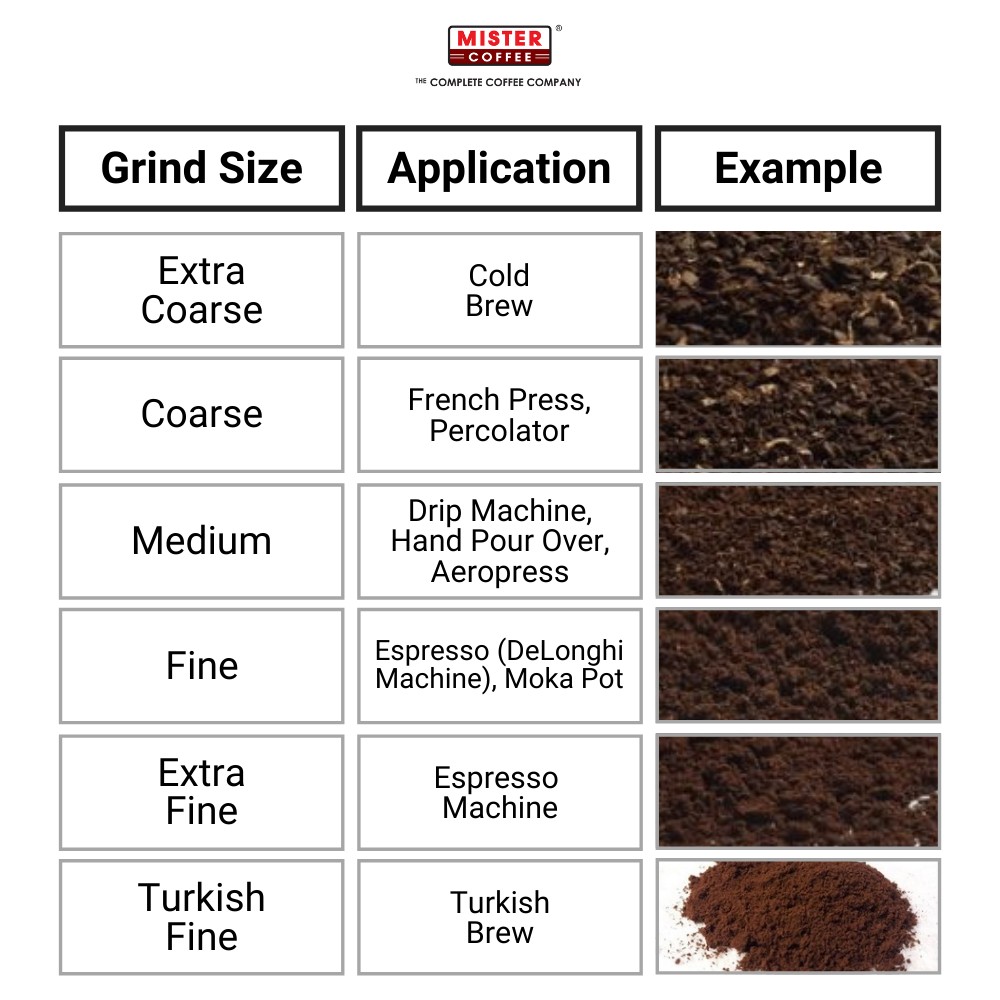This infographic, prominently featuring the red and black logo of Mr. Coffee with the tagline "Complete Coffee Company," provides a detailed guide on coffee grind sizes and their recommended applications. Below the logo, the infographic is divided into three main columns. The first column lists various grind sizes in bold black text, ranging from "Extra Coarse" to "Turkish Fine." The second column, also in bold text, corresponds with the grind sizes, detailing their applications such as "Cold Brew," "French Press," "Drip Machine," "Espresso," "Espresso Machine," and "Turkish Brew." The final column offers visual examples, featuring actual images of coffee grounds progressing from extra coarse to the finest Turkish grind. This clear and informative chart serves as a useful reference for coffee enthusiasts, matching each grind size with its optimal brewing method.